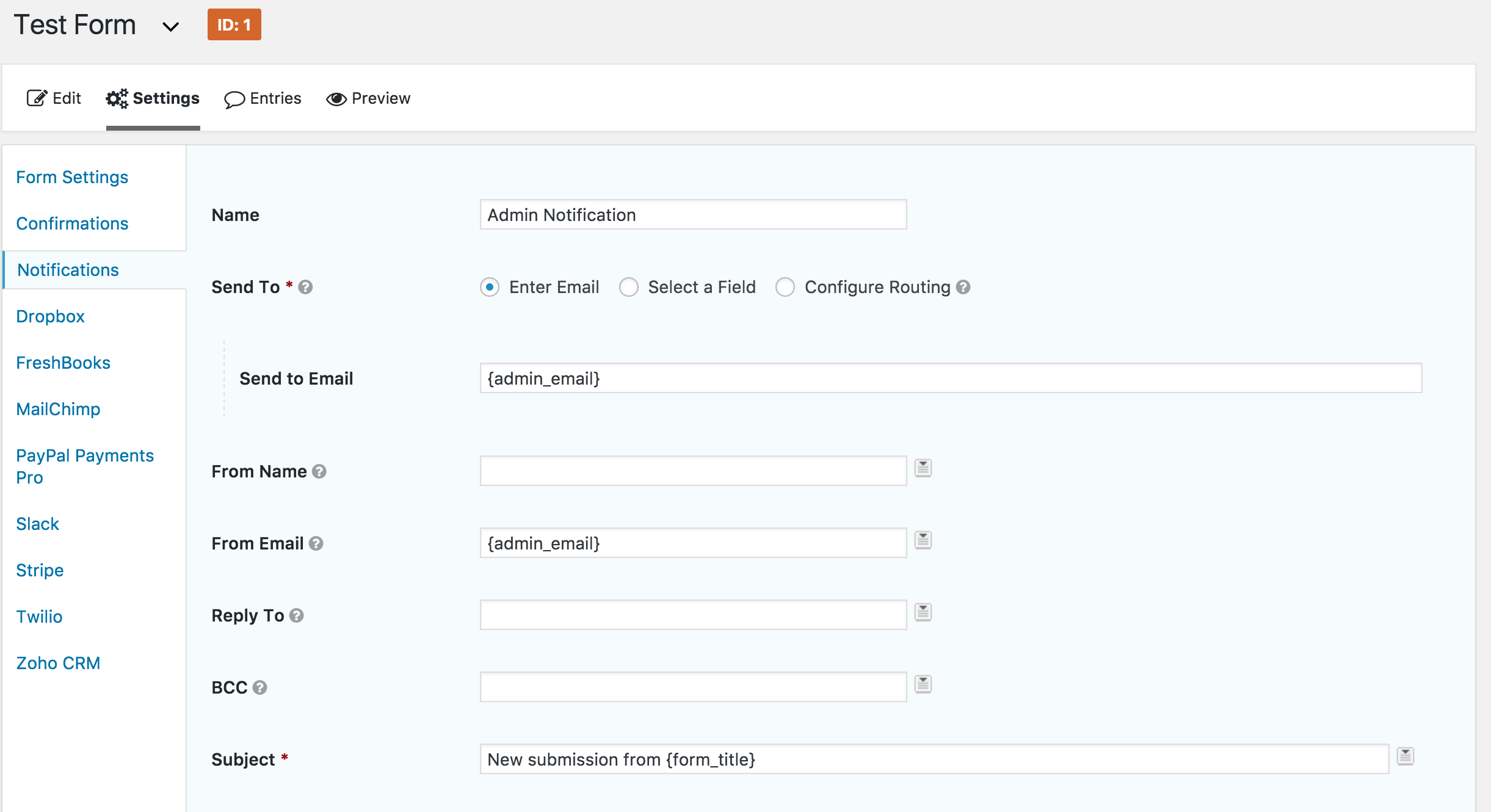The image contains a user interface from a form management application.

At the top, there's a light gray bar featuring black text on the left that reads "Test Form," accompanied by a black downward arrow to its right. Adjacent to these is an orange button with white text that says "ID: 1."

Below this bar, on the left side, there is a white navigation menu with black text featuring several clickable options: "Edit," "Settings," "Entries," and "Preview," each with a small icon to their left. "Settings" appears to be selected since it's underlined.

Further down on the left, there are additional options written in blue text: "Form Settings," "Confirmations," "Notifications," "Dropbox," "FreshBooks," "MailChimp," "PayPal Payments Pro," "Slack," "Stripe," "Twilio," "Zoho CRM." The "Notifications" option is selected.

On the right side of the image, within the "Notifications" section, there are several input fields and settings. The first field is labeled "Name," and contains the text "Admin Notification." Below this is the "Send To" section, where the user can choose from "Enter Email," "Select a Field," and "Configure Routing." It is currently set to "Send To Email," with a text box underneath containing "Admin Email."

Following this, there are more input fields: "From Name" with an empty text box, "From Email" with "Admin Email" pre-filled, "Reply To" with an empty text box, "BCC" with an empty text box, and "Subject," which has a text box containing the text "New Submission from Form Title."